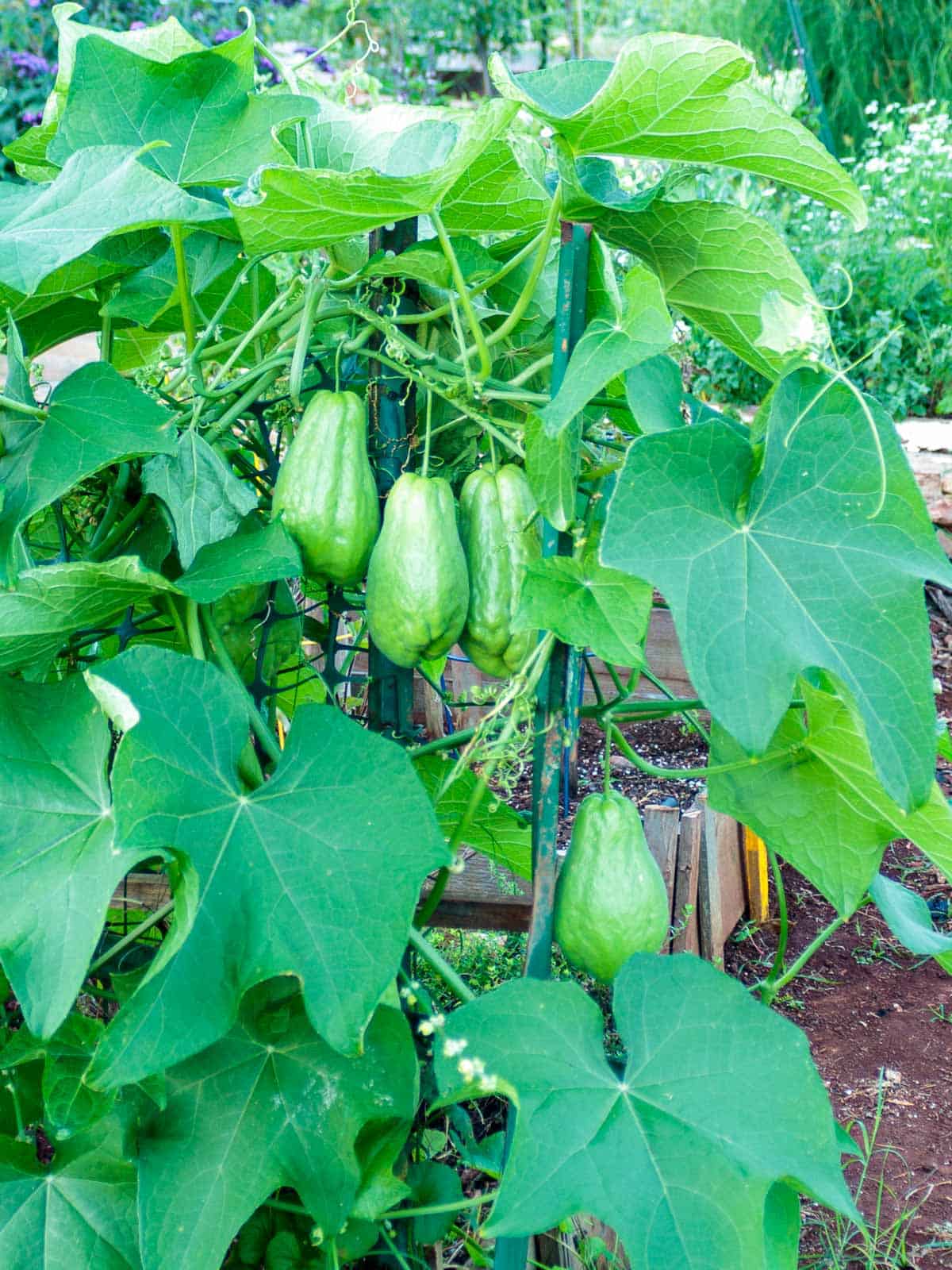This is a vibrant outdoor color photograph, taller than it is wide, showcasing a lush green plant dominating the foreground. The plant is supported by a wooden trellis and features large, wide leaves that resemble those of lily pads, some with four distinct points. Nestled among these expansive leaves are four light green, pear-shaped fruits or vegetables, hanging from thick green stems. The strikingly green hue of the plant contrasts with the brown soil visible in the bottom right corner. In the background, beyond the plant, a faint view of a fence is discernible along with small white flowers dotting the scene. A curious small stripe of yellow is partially hidden behind one of the leaves, adding another element of intrigue to the image. The overall composition highlights the lushness and richness of the plant, capturing the essence of thriving growth.